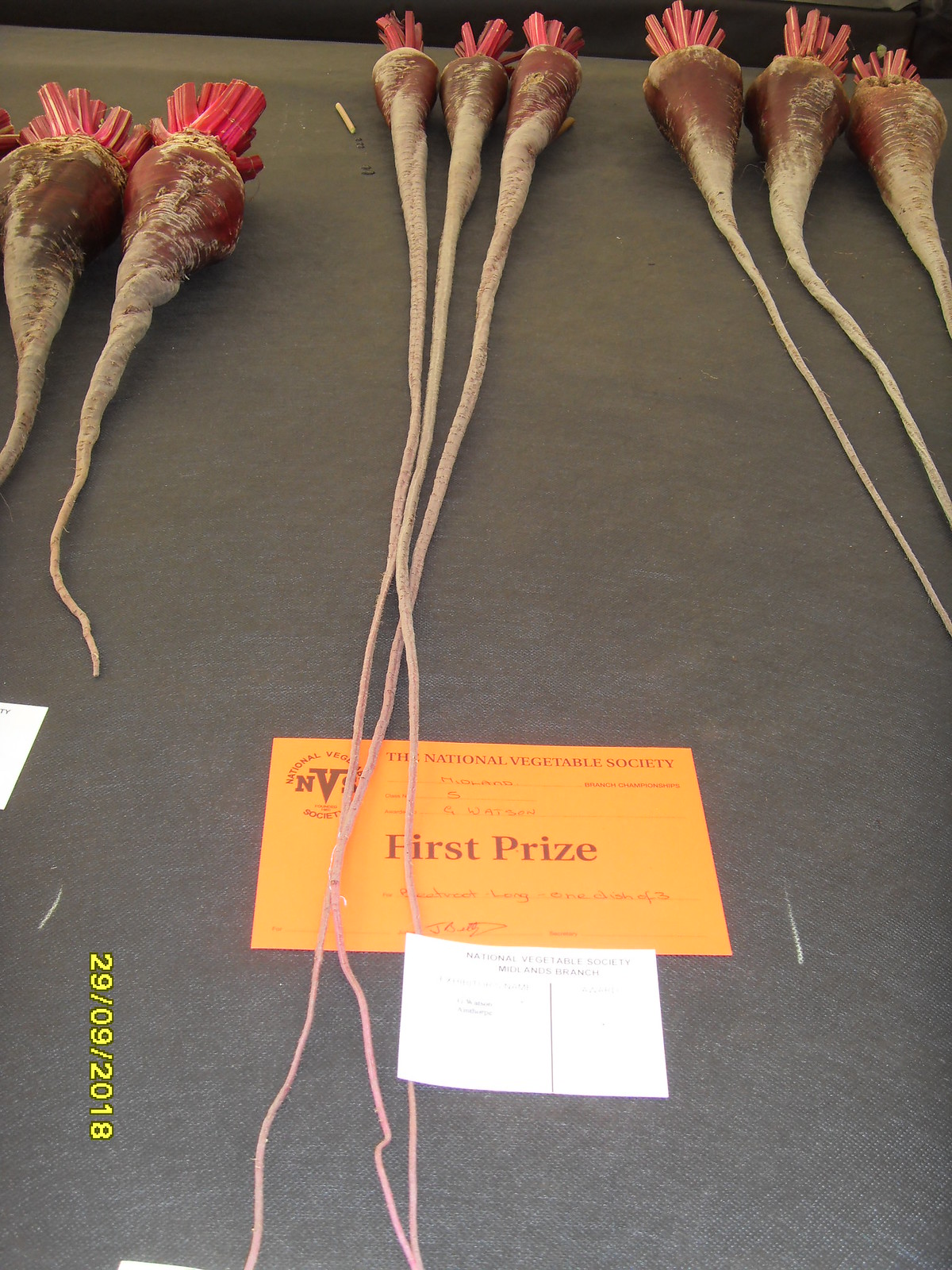The photograph portrays eight red vegetables, which appear to be radishes, arranged on a gray table. They are segmented into three groups: two plump radishes on the left, three elongated ones in the middle, and three slightly broader elongated radishes to the right. Each vegetable has a triangular shape with long roots and red stalks at the top. An orange sign at the center beneath the middle group reads, "National Vegetable Society First Prize," with additional smaller, unreadable text. A white sign beneath it appears to belong to the National Vegetable Society, also featuring small, blurry text. At the bottom left corner, the date "29-09-2018" is printed in yellow, running sideways. The photograph is characterized by rich colors, including gray, yellow, red, maroon, orange, and white, suggesting a vibrant presentation likely from a vegetable contest possibly held outdoors.